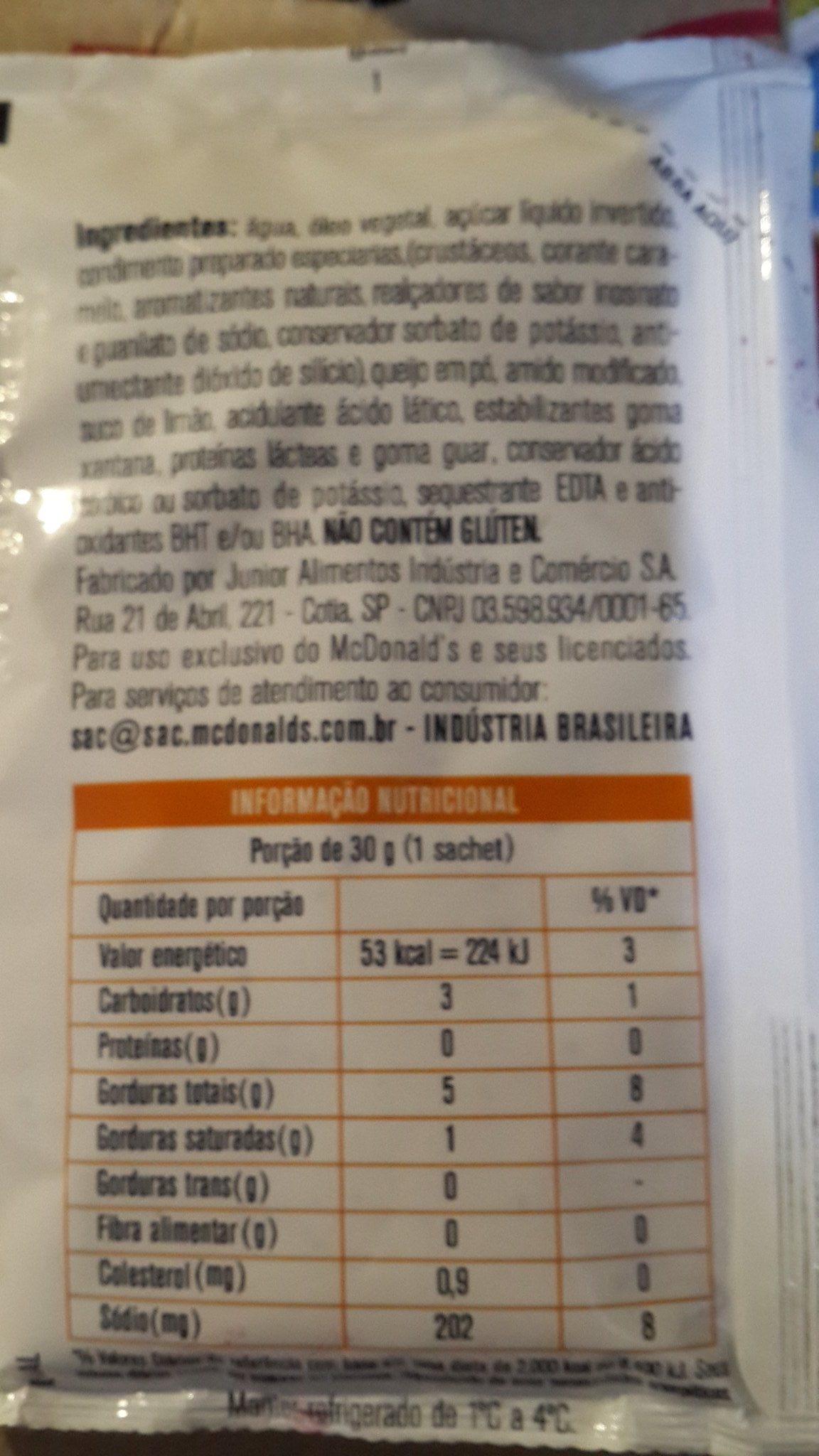This is a detailed and close-up yet blurry photograph of the back of a shiny white plastic package from McDonald's, possibly a food or sauce packet from Brazil. The top of the package features an ingredients list in Portuguese, including items like "agua" (water) and "oléo vegetal" (vegetable oil), along with the statement "não contém glúten" (no gluten). The package also displays nutritional information under the header "Informação Nutricional" in an orange box with a grid. The ingredients and nutritional details are printed in black letters and numbers. The grid shows nutritional values such as "53 kcal = 22 kj," and other figures likely relevant to protein, carbohydrates, and fats. An email address "sac.mcdonalds.com.br" indicates the product is from McDonald's Brazil.